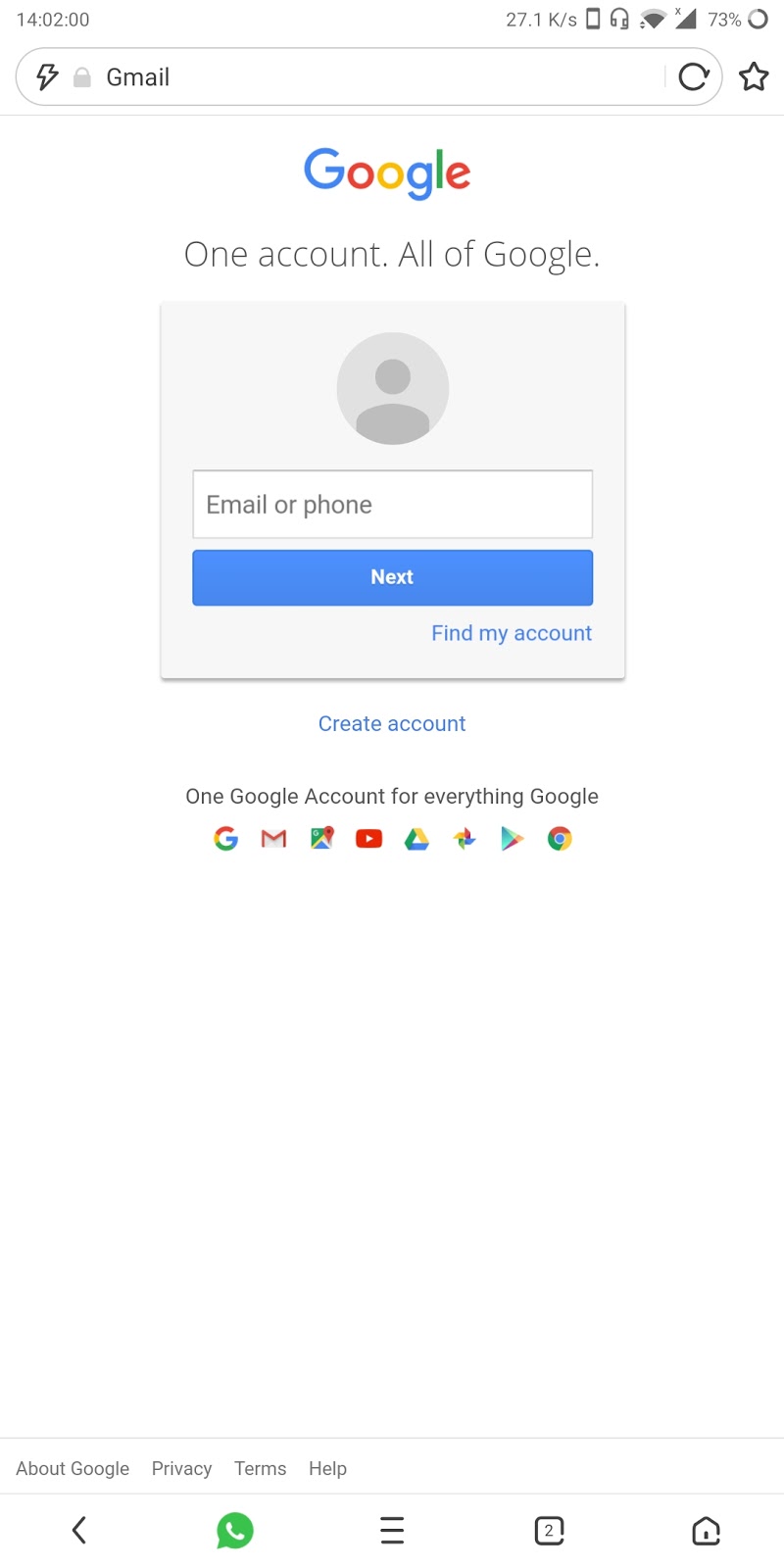A detailed screen capture of a smartphone displaying the Gmail login page. The device shows the time as 14:02 and its battery is 73% charged. Dominating the screen is the Gmail app interface. At the top, the "Gmail" title is prominently displayed, followed by the iconic colored letters spelling out "Google" with the tagline "One account. All of Google." Below this, there is a text box labeled "Email or phone" indicating users can enter either their email address or phone number to sign in. 

Below the text box, there are two buttons: "Next" for proceeding with the login process, "Find my account" for account recovery, and "Create account" for new users.

Towards the bottom of the screen, it reiterates the message with the text "One Google Account for everything Google." There are various colored icons symbolizing different Google services and apps. Additionally, the lower part of the screen provides more links including "About Google," "Privacy," "Terms," and "Help." There are also navigation icons like a back button and a phone button.